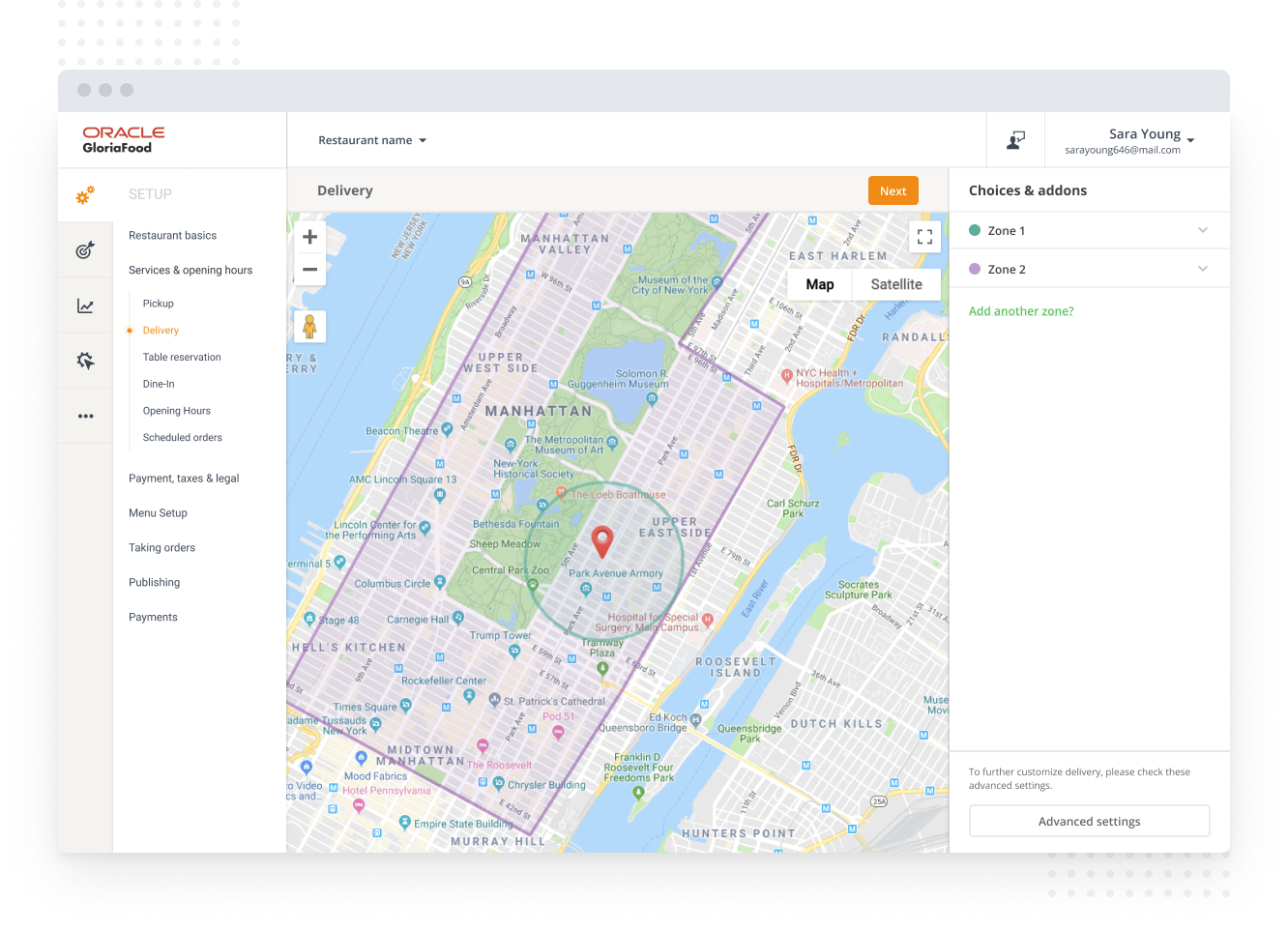The image depicts a webpage dedicated to map settings, likely for a food delivery service. The top banner serves as the header and appears in light gray, featuring three ellipses on the right. To the left and directly below the banner, the page includes the Oracle Gloria Food logo, with "Gloria Food" presented as a single word.

Below the logo, there is a navigation menu categorized under "Setup." This section comprises several subsections: "Restaurant Basics," "Services and Operating Hours," which further includes "Pickup," "Delivery" (highlighted in yellow), "Table Reservations," "Dine-In," "Scheduled Orders," "Payments, Taxes, and Legal."

Adjacent to this menu is a detailed list of options under "Menu Setup," "Taking Orders," "Publishing," and "Payments."

To the right of these sections, the restaurant's name is displayed alongside a drop-down arrow for selection purposes. Below this, framed by a gray border, is the "Delivery" section, containing various settings. Positioned on the extreme right edge of the gray border is an orange "Next" button.

Below the section header, the user is identified as Sarah Young, with an email address of sarahyoung646@gmail.com. Underneath this, there is a panel for choices and add-ons featuring a green dot labeled "Zone 1" with a drop-down arrow, and a purple dot labeled "Zone 2" also with a drop-down arrow. Additionally, there's an option to "Add another zone."

At the bottom of this section, there is an invitation to "further customize delivery" with a button labeled "Advanced Settings" for more detailed configurations.

The map indicates the location as the Park Avenue Armory, situated in upper Manhattan, where Oracle Gloria Food's services are presumably available.